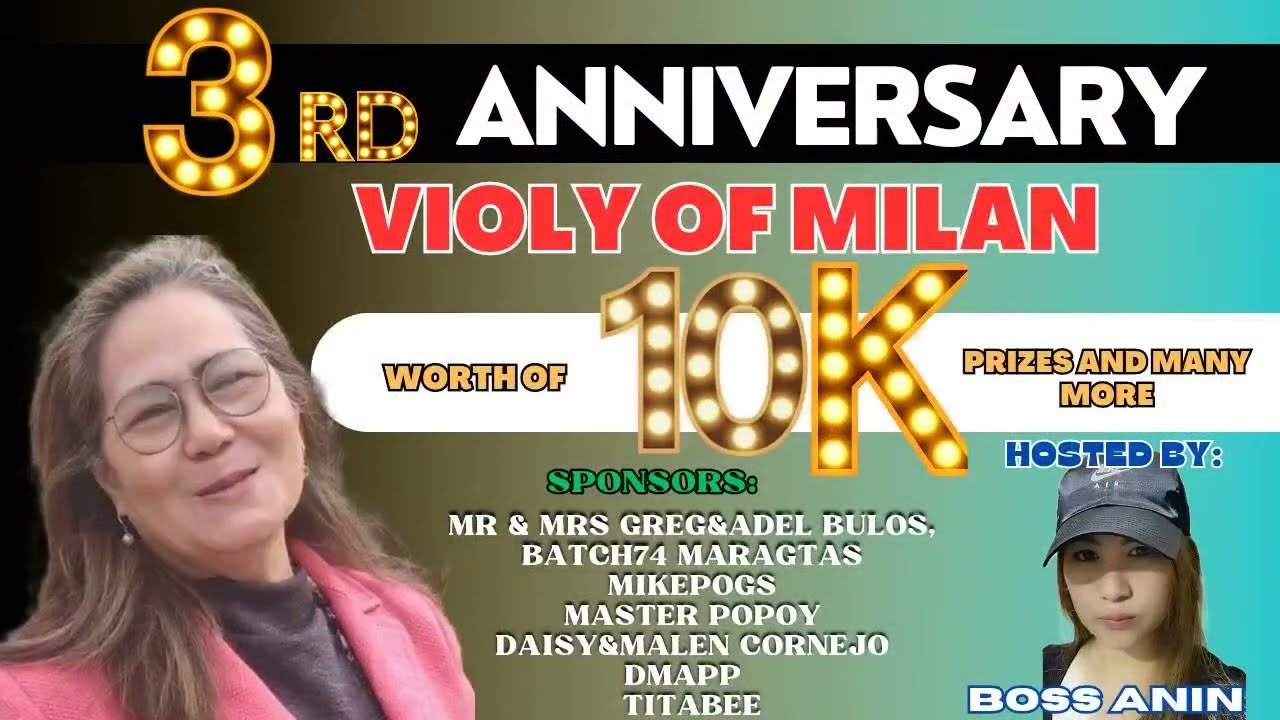This vibrant and detailed collage graphic celebrates the third anniversary of the Viola of Milan. Dominating the top portion of the image is a black banner featuring the words "Third Anniversary." The word "Third" is stylized in a flashy Las Vegas-style marquee font, with bright gold lights, while "Anniversary" is written in bold white block letters. Below this, the name "Viola of Milan" is prominently displayed in striking red text. 

A white banner extends from the right side, announcing "worth of 10K prizes and many more" in gold text, with "10K" also styled in the distinctive gold-lettering and white light treatment. 

On the lower left, there is a head-and-shoulders photo of an older woman, possibly in her 50s, wearing a pink jacket over a gray shirt and round glasses. She has shoulder-length brown hair, graying slightly, and tilts her head to the left, smiling gently. 

On the right, another woman is depicted with the label "hosted by Boss Anine." She appears younger, wearing a black Nike Air baseball cap and a black jacket, and looks directly at the camera with a serious expression.

Centered near the bottom, the word "Sponsors" is highlighted in green, followed by a list of names in white text: Mr. and Mrs. Greg and Adele Boulus, Batch 74 Maragatas, Mike Poggs, Master Popoy, Daisy and Malen Cornejo, DMAP, and Titibi.

Overall, the image is a vibrant and introspective advertisement highlighting various elements that collectively celebrate the significant milestone of Viola of Milan's third anniversary.